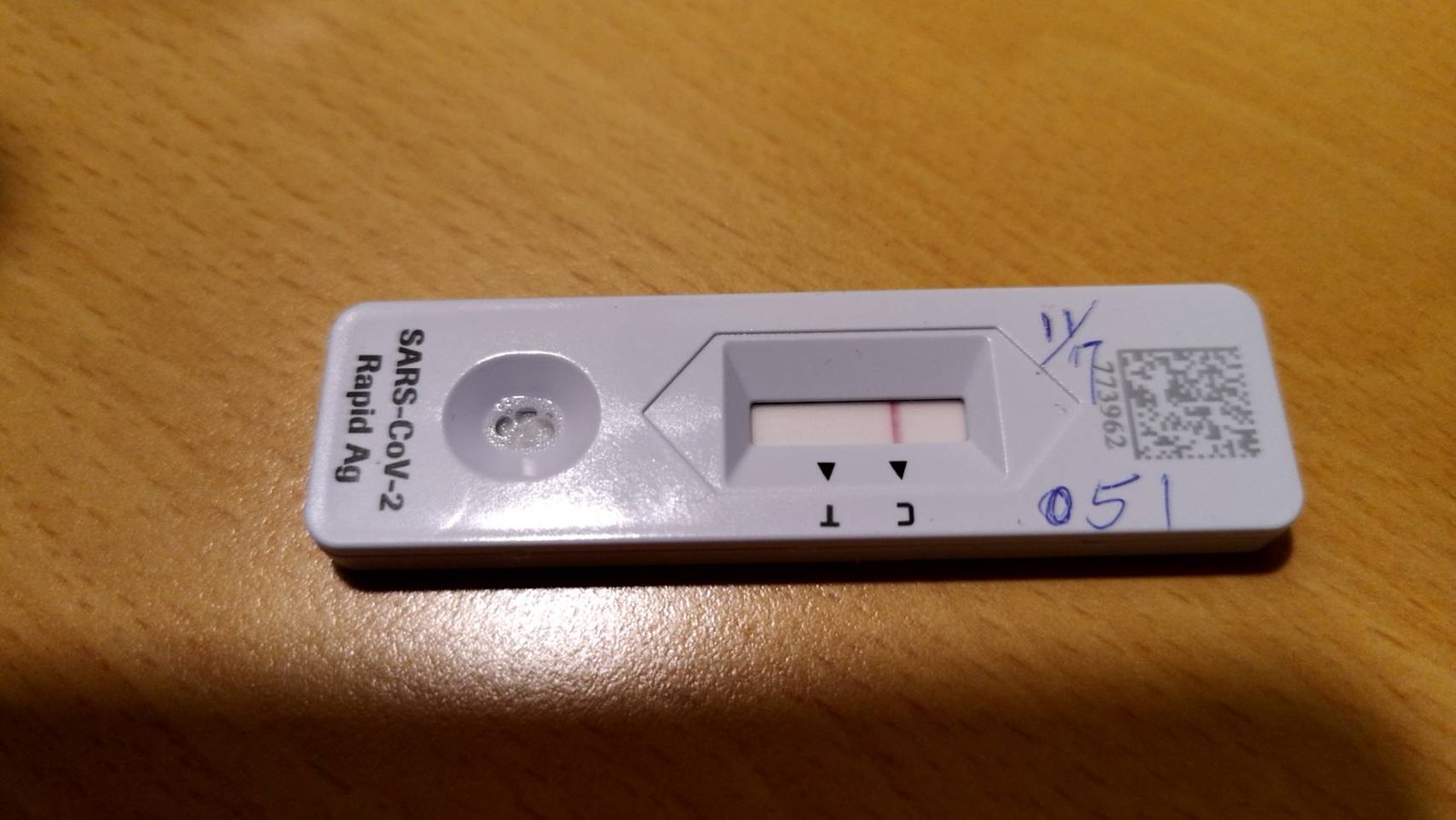In this image, we see a COVID-19 rapid test kit placed on a light brown desk. The test kit appears upside down. The kit itself is a white rectangular piece of plastic with a matte finish. On the right side of the kit, there is a QR code with some numbers printed below it. Over these numbers, someone has written "11/7" and "051" with a blue ink pen. 

The test kit features a diamond-shaped pattern, and within this pattern is a small gray screen displaying a single red line located beneath the letter "C." To the right of this, there is another section labeled "T," which remains blank. Additionally, there is a small hole on the left side of the kit.

At the bottom of the test strip, or on the left side when viewed in its current position, the label "SARS-CoV-2 Rapid AG" is printed in black text.